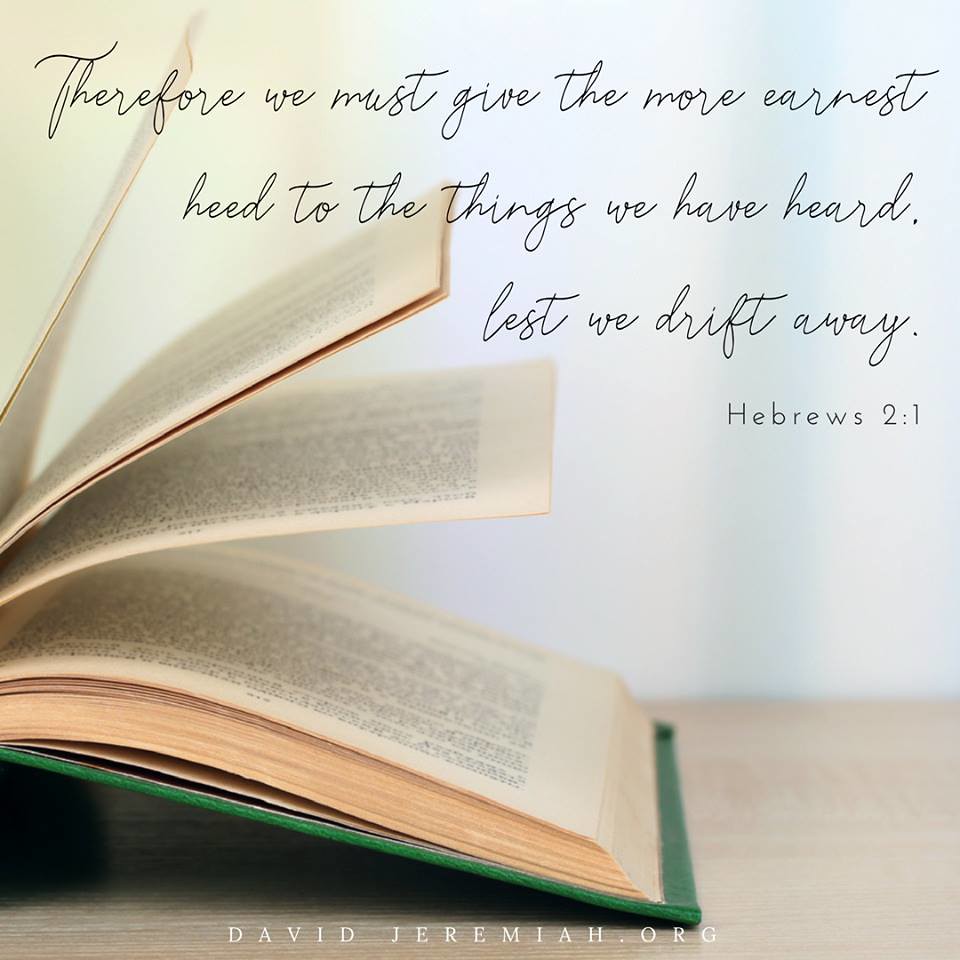The image features an open, slightly aged book with a green cover, lying on a light brown wooden table. The pages, some standing upright as if caught in a breeze, are white with a beige tint. A quote in black cursive overlaying the image reads, "Therefore, we must give the more earnest heed to the things we have heard, lest we drift away," followed by "Hebrews 2:1" in regular black font. The background, which appears out of focus, transitions from light blue to a pale yellow, suggesting the presence of a window with light filtering through. At the bottom of the image, in all-capital white lettering, it says "DavidJeremiah.org."